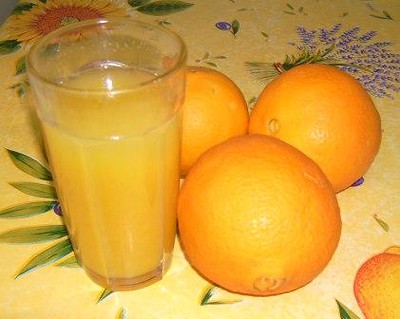This color photograph captures a beautifully arranged still-life scene on a beige-yellow table adorned with floral designs, prominently featuring a sunflower and bundles of purple lavender with green leaves. At the center of the composition are three large, bright navel oranges, arranged in a triangular formation, with their vibrant orange hues creating a striking visual contrast against the table's floral background. The light source, seemingly from the viewer's perspective, casts soft highlights on the oranges and reflects off their slightly dented surfaces, adding depth and texture to the image.

To the left of the oranges stands a tall, clear glass filled almost to the brim with light, pale orange juice. The glass features faint vertical ridges that catch the light, further enhancing the photograph's intricate details. The cohesive interplay of color and light, alongside the carefully chosen arrangement of oranges and juice, brings a sense of freshness and vibrancy to the scene, making it a visually captivating and detailed composition.